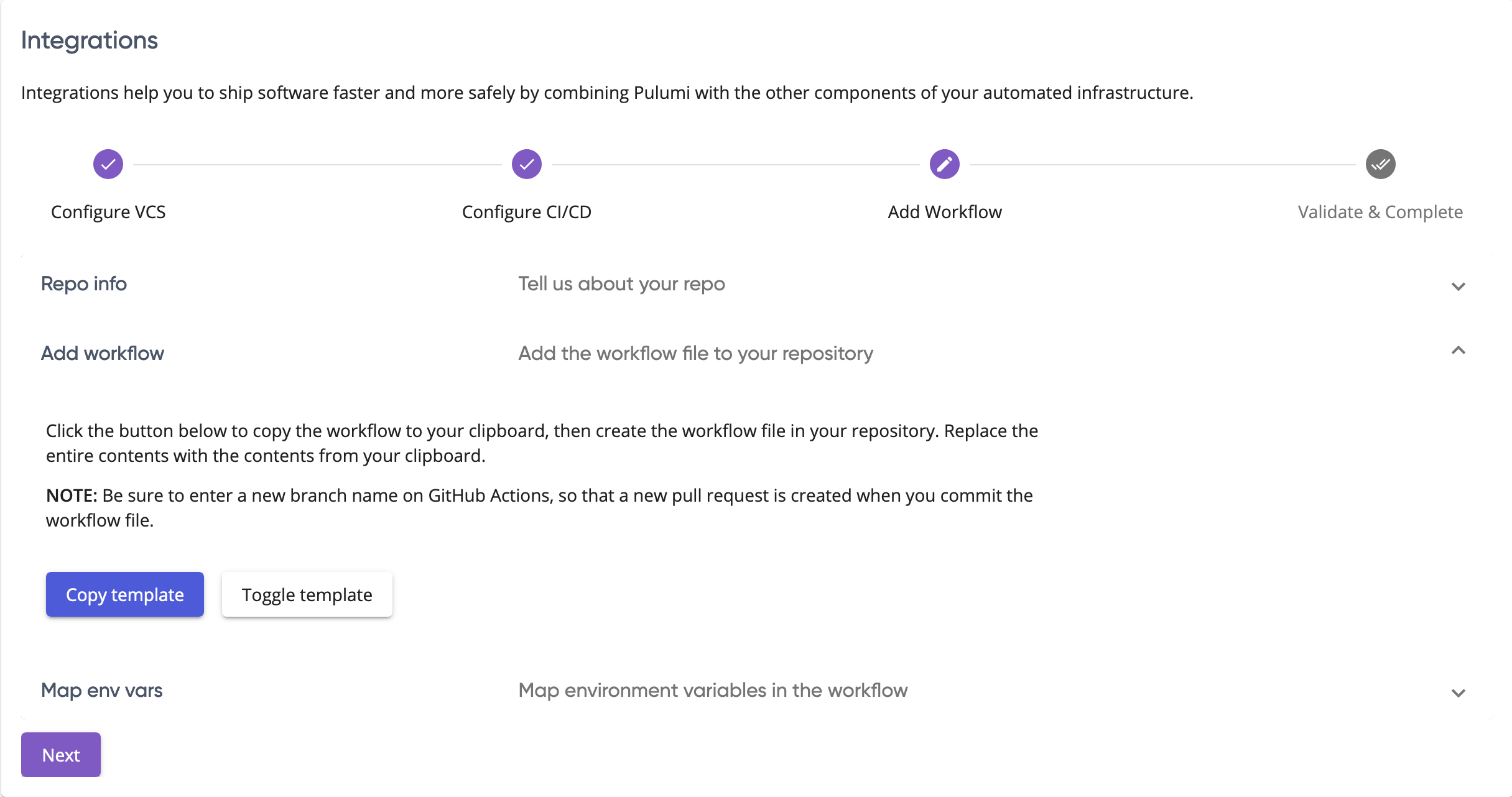This image depicts a section labeled "Integrations" on a web page, which highlights how integrations aid in shipping software more quickly and safely by combining Pulumi with various components of your automated infrastructure. Below the main section, the text explains steps for setting up integrations: 

- Configure your VCS (Version Control System)
- Configure CI/CD (Continuous Integration/Continuous Deployment)
- Add Workflow
- Validate and Compare

To the left, there's a detailed step-by-step guide under "Tell us about your repo info," which instructs users on how to integrate their repository with the provided tools. It prompts the user to click a button to copy the workflow to their clipboard and then create the workflow in their repository. The visual layout includes explanatory text and actionable steps, making it user-friendly for developers aiming to streamline their coding and deployment processes.